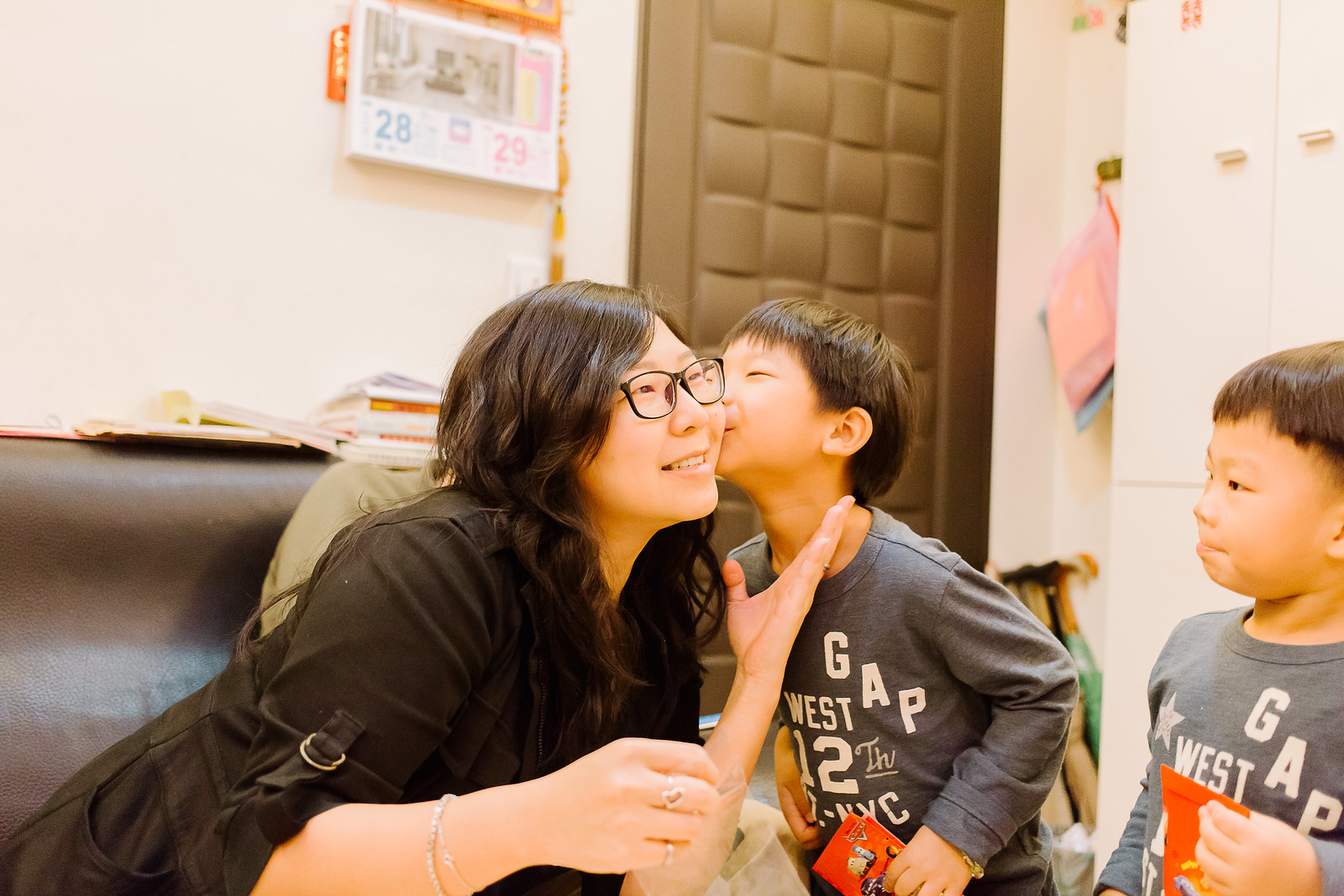The image captures a heartwarming moment between an Asian woman and two young boys, likely her sons, in what appears to be a classroom or a family-friendly interior setting. The woman, in her twenties or early thirties, has long dark brown hair cascading down the sides of her face and wears dark-rimmed glasses. She is dressed in a brown coat, and beneath it, she may have a black shirt or dress. She has a slight, gentle smile as one of the boys leans in to kiss her left cheek. She tenderly reaches up with her right hand to touch him, displaying a few rings and bracelets on her hand and wrist.

The boys, who have similar short, bowl-like haircuts and are wearing matching gray long-sleeved shirts with "GAP" written in white letters, appear to be the same age and could be twins. They each hold orange cards and have friendly, slightly mischievous smiles. The boy who is not kissing the woman stands to the right, gazing at her with affection.

The setting includes a dark brown leather bench situated in the top left and bottom left corners, an orange padded doorway area in the background, and hooks on the wall suggesting it might be a school. A calendar, some books, and other items provide additional context, creating a cozy and lived-in atmosphere.